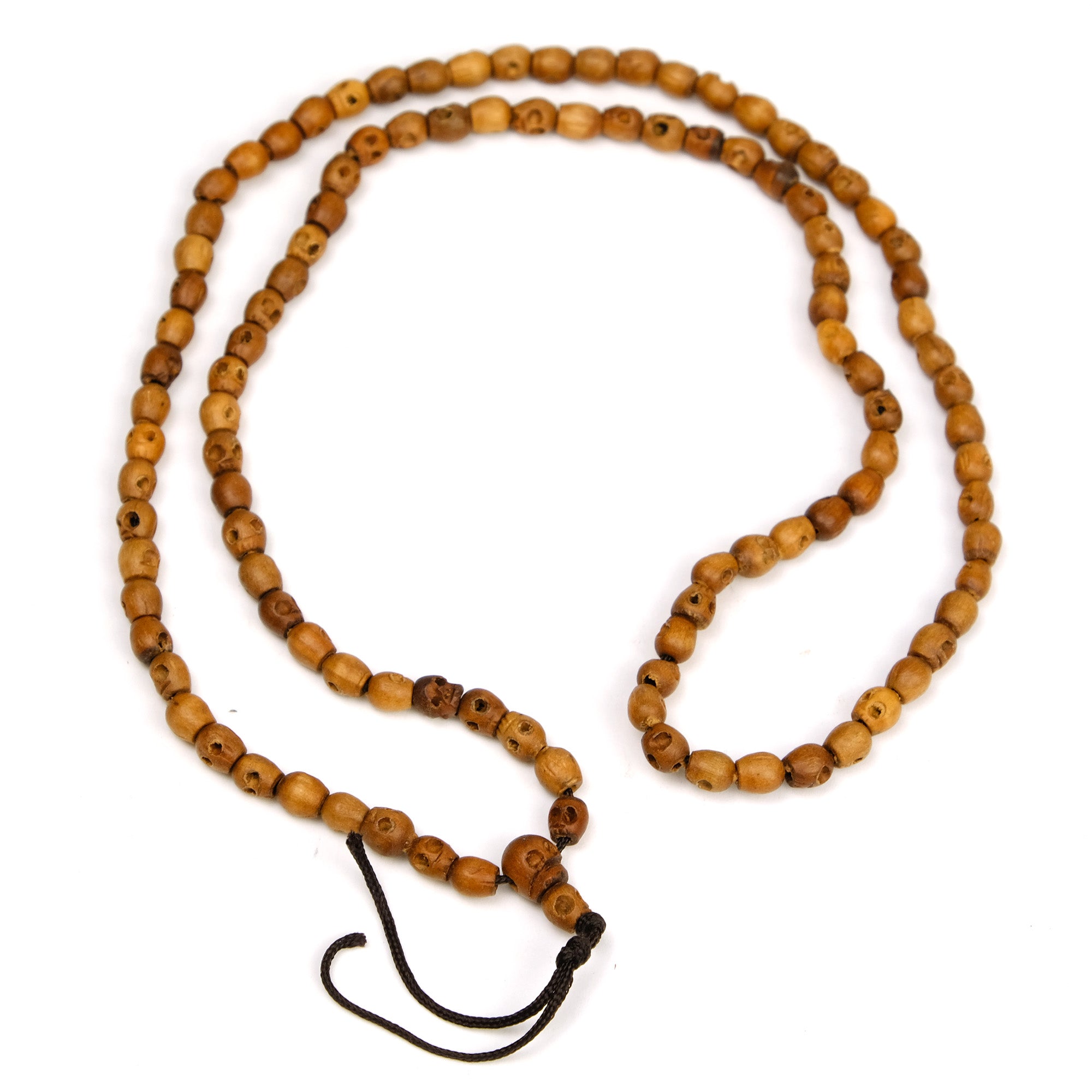The image showcases a close-up of an ancient-looking necklace that occupies the entire frame, set against a stark white backdrop. The necklace, possibly made of handcrafted wooden beads, is intricately tied with what appears to be a black suede string. The beads, though uniformly sized, exhibit a variety of shapes and textures, ranging from rounded to somewhat squarish forms. They come in different shades of brown and tan, some adorned with tiny black spots, suggesting age or weathering over time. The beads are designed to resemble tiny skulls with detailed faces, adding a unique and potentially historical character. Spread out and possibly long enough to be doubled, the necklace appears to be well-crafted, almost museum-worthy, with each of the estimated 100 beads contributing to its detailed and intricate layout.